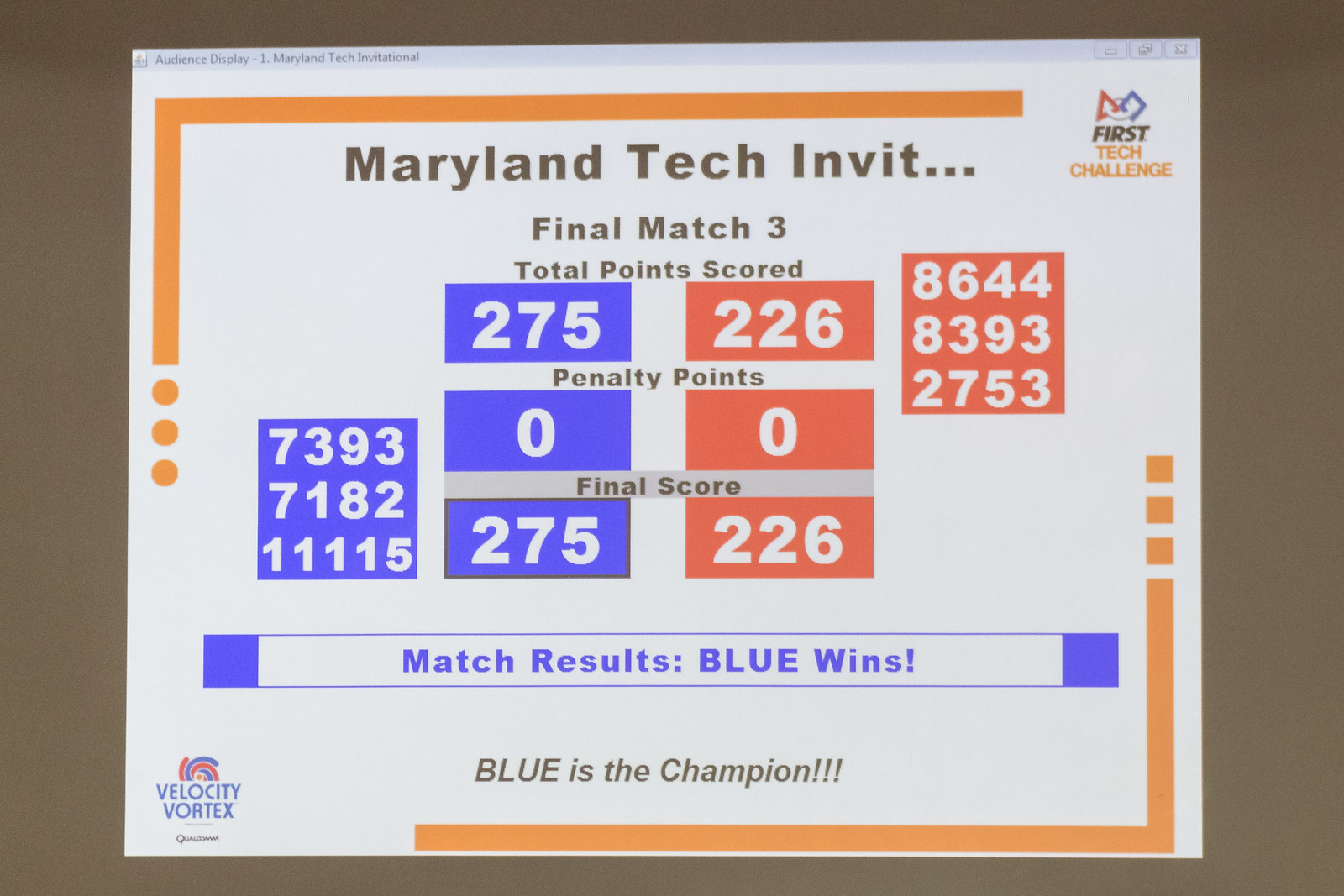This photograph captures a rectangular poster attached to a brown surface, featuring details of the Maryland Tech Invite Final Match 3. The poster has a white background with black text. At the top, a light blue horizontal strip resembling a window screen highlights the event title: "Maryland Tech Invite Final Match 3 Total Points Scored." Below this, on the left, blue-colored boxes display the score "275," and on the right, red-colored boxes show the score "226." Underneath, it reads: "Penalty Points 0-0. Final Score 275-226. Match Results: Blue Wins. Blue is the champion." The term "Blue" is notably capitalized. In the top right corner, the logo for "First Tech Challenge" is visible, and in the bottom left corner, another logo is present with the text "Velocity Vortex." Orange lines appear at the top and bottom of the poster, suggesting it might be a screenshot or a photo taken from an overhead projector.